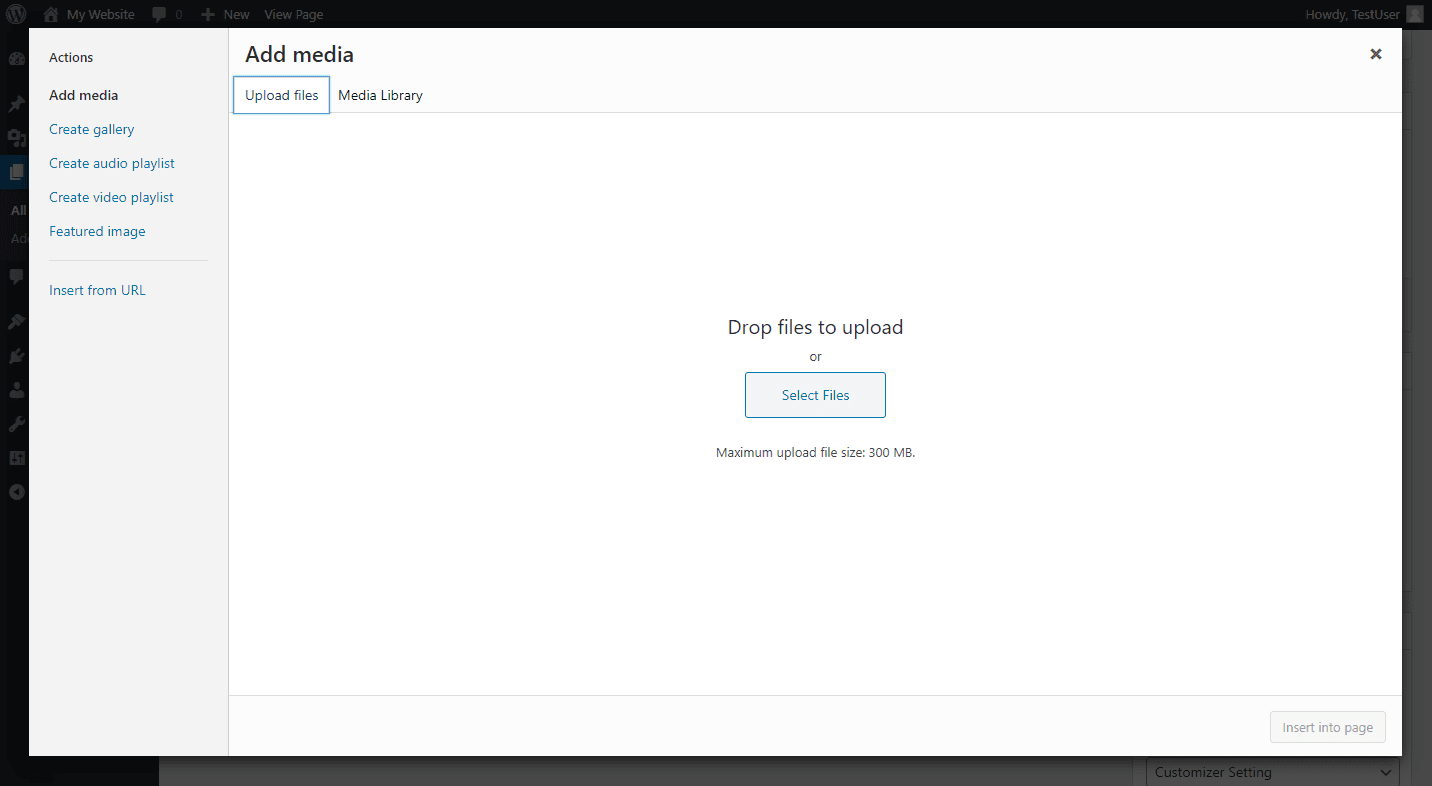This is a screenshot from the settings menu on a computer, displaying options for managing media content. 

On the left side, there is a vertical column with several links labeled as follows: "Actions," "Add Media," "Create Gallery," "Create Audio Playlist," "Create Video Playlist," "Featured Image," and "Insert from URL." 

On the right side of the screen, the user has selected the "Add Media" option. Under the "Add Media" section, there are two main tabs: "Upload Files" and "Media Library." The user is currently in the "Upload Files" tab. Here, the interface provides the option to either drag and drop files into an outlined area or click a button labeled "Select Files" to manually choose files from the computer. The maximum upload file size is indicated as 300 megabytes. Once a file is uploaded or selected, there is an option in the bottom right corner to "Insert into Page," which facilitates adding the chosen media files to a webpage.